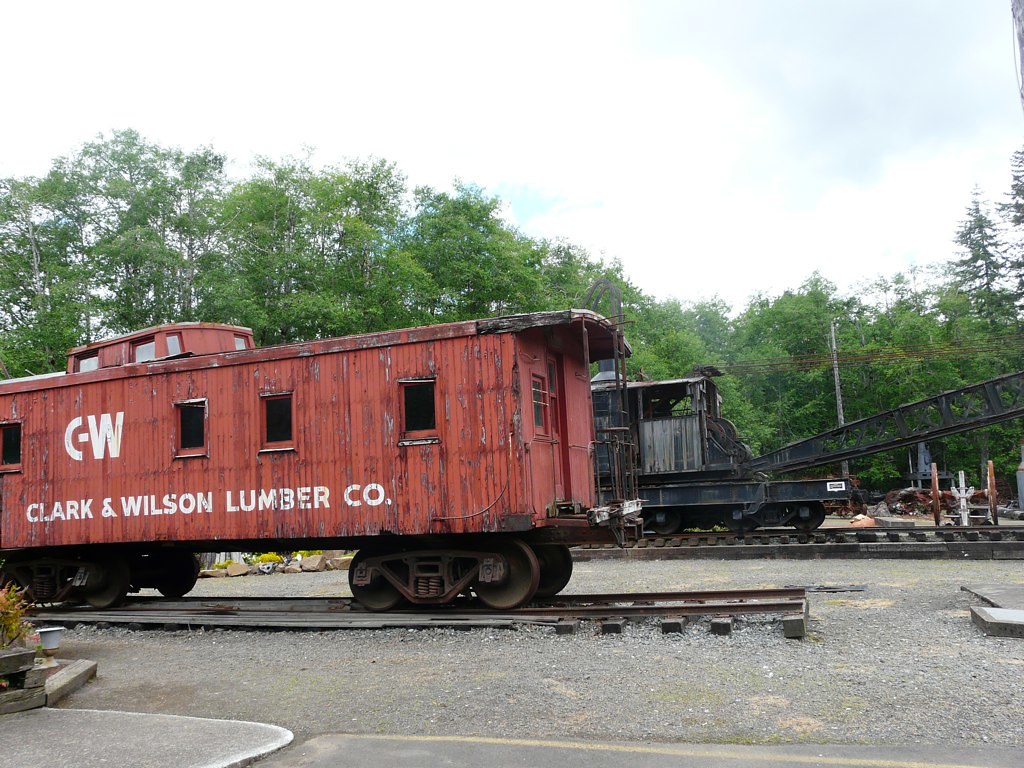The photograph captures a nostalgic scene in a rail yard featuring an aged, red wooden train car, with faded paint giving it a slightly brownish hue in places. The car prominently displays white lettering reading "C-W" and "Clark and Wilson Lumber Company" on its side. Resembling an old caboose, it boasts four visible windows and a rear door, and rests on rusty, disused tracks that abruptly end to the right of the frame. The ground beneath consists of both concrete and gravel, providing a rugged consistency to the setting.

In the background, there's an indistinct black train car, possibly equipped with a crane, indicating its industrial past. This secondary car is only partly visible, revealing the complexity and history behind it. Towering, lush green trees frame the entire scene, adding to the rustic charm of the vintage rail cars. The light blue sky, dotted with white clouds, lends an almost ethereal brightness to the image, evoking a sense of serenity and timelessness. No people are present, leaving the scene tranquil and undisturbed.